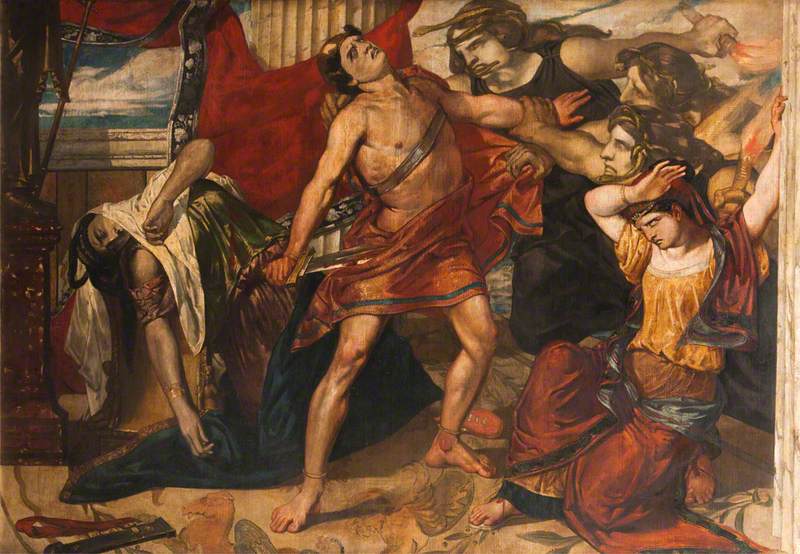The painting, likely from the Roman era, depicts a dramatic battle scene centered around a mostly naked man clad in a red wrap around his waist. Positioned in the center, the man stands with his head thrown back and eyes closed, seemingly in a moment of intense emotion. His left hand clutches a large, bloody dagger, while his right hand is being grasped by an attacking figure. The focal man has black hair and is portrayed in a moment of significant strain.

To the man's left, a woman in a white robe and green dress with a brown skirt lays draped over a couch, seemingly dead from the stab wound inflicted by the central figure. Her left arm is crossed over her chest, and her right arm hangs limply to the ground. Above her, there is a background painting of a blue sky and water.

On the right side of the composition, a cluster of figures in varying states of distress look towards the central man. One of these figures, clad in black, grabs the man's left arm, while another person, visible only by their head adorned with flowers, also restrains him. A woman towards the bottom, with her arm raised as if shielding herself, adds to the chaotic scene.

Further to the right, another woman lies on the ground with her arm raised overhead, reaching towards a pillar adorned with a torch or similar object. Behind these characters, there are flags and drapery adding depth to the scene. The overall composition—with its array of distressed figures, dynamic positioning, and classical elements—recounts a vivid and violent moment steeped in historical artistry.